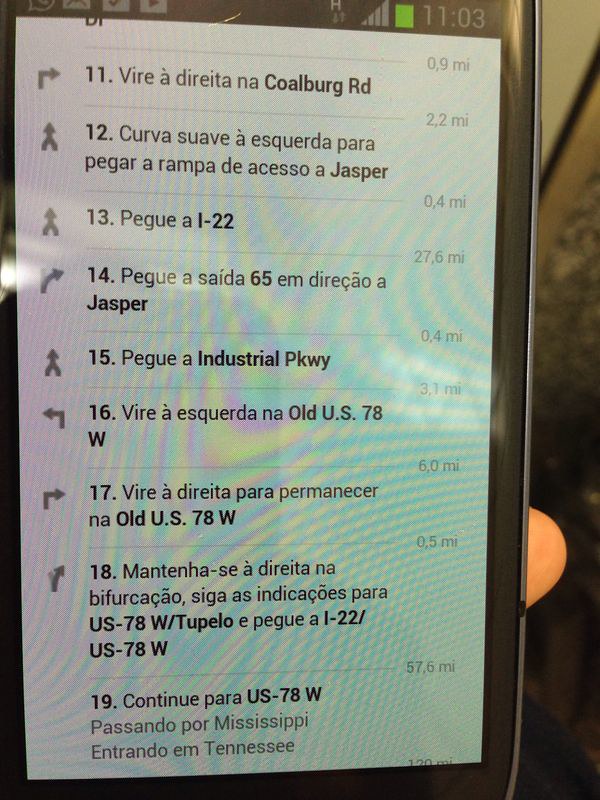A printed set of MapQuest directions is depicted, showcasing a translated route in Spanish for an American journey. The itinerary begins at Step 11 on Colberg Road and concludes at Step 19, instructing users to continue on US 78 West. The route traverses from Mississippi and appears to include an entrance into Tennessee, indicative of a cross-state journey within the United States. The directions are detailed and comprehensive, ensuring a clear path for the traveler.